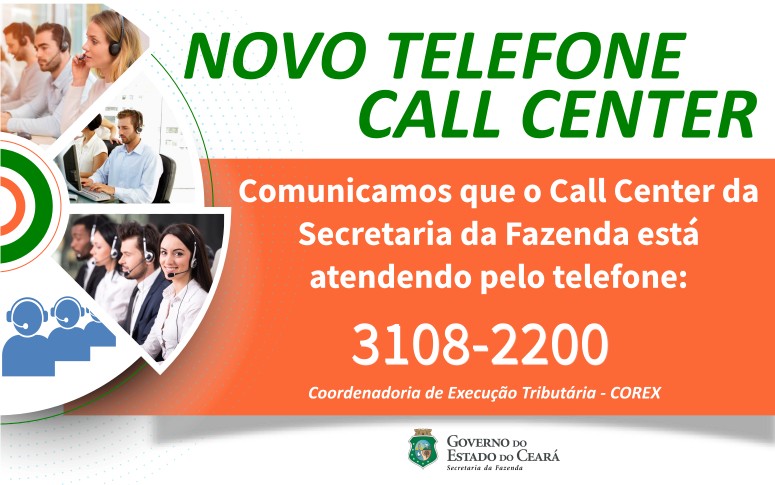The image appears to be an advertisement for a call center, likely in Spanish. The card has a rectangular layout, divided into two main sections: the bottom section is orange with white text, while the upper section is narrower with a white background and green text. On the left side of the card, there is a semi-circle featuring various images of people working in a call center, including three photos of actual humans wearing headsets and interacting with customers, and one with blue cartoon figures. Inside the semi-circle, there is a green and orange bullseye, matching the card's color scheme. The text at the top of the card reads, "Nuevo Telephone Call Center," and the middle section states, "Comunicamos que el call center de la Secretaría de Hacienda está atendiendo el teléfono 3108-2200." The bottom section includes a green badge or coat of arms and mentions, "Gobernador del Estado de Sera." Based on the text, this appears to be an official notice or advertisement for a call center associated with the Secretaría de Hacienda, including contact information and government affiliation.